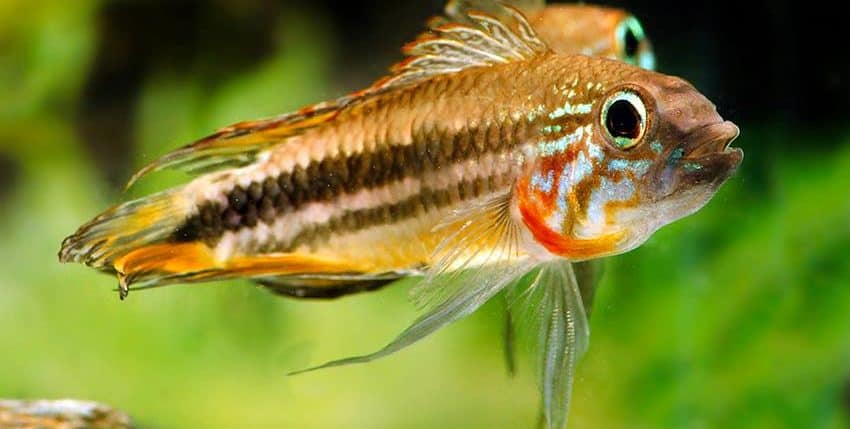The image captures a close-up of two small, teardrop-shaped fish in an aquarium. The fish in the forefront has a rounded head and a more pointed tail, its scales revealing intricate patterns. Predominantly brown, it features a dark brown and gray stripe running down its side, along with silver markings on its face. The fish’s large, silver eyes with black pupils are prominent, and its semi-translucent fins stretch along the top and bottom of its body. Around its gills, an orange hue stands out, contrasting with the slightly open brown lips. The fish also displays a sunburst pattern of orange and white around its eye, and a series of dark stripes crossing its body. In the blurred background, another nearly identical fish can be seen, though mostly obscured. The backdrop of the image is filled with out-of-focus green aquarium plants, contributing a soft, greenish tint behind the clear water. The detailed textures and colors of the fish’s scales, fins, and facial features are especially vivid in this close-up photograph.